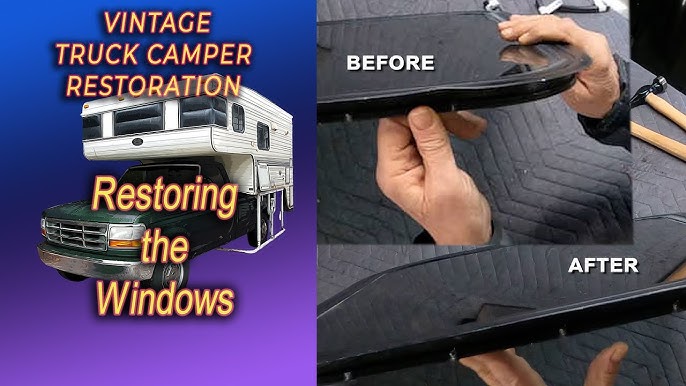The advertisement image is divided into two main sections. On the left-hand side, which fades from blue at the top to purple at the bottom, there's a green pickup truck with a vintage camper attached. The text in yellow bubble lettering reads "Vintage Truck Camper Restoration" followed by "Restoring the Windows". The right-hand side showcases a before-and-after sequence. The top image, labeled "before" in white letters, displays a man's hands—dressed in a long-sleeve shirt—holding a window with a bent frame. The bottom image, labeled "after", shows the same hands holding the now-straightened window. Below the window, there's a gray pad on a brown table, with two hammers visible—one with a black top. The overall background and side-by-side layout emphasize the restoration process of vintage truck camper windows.